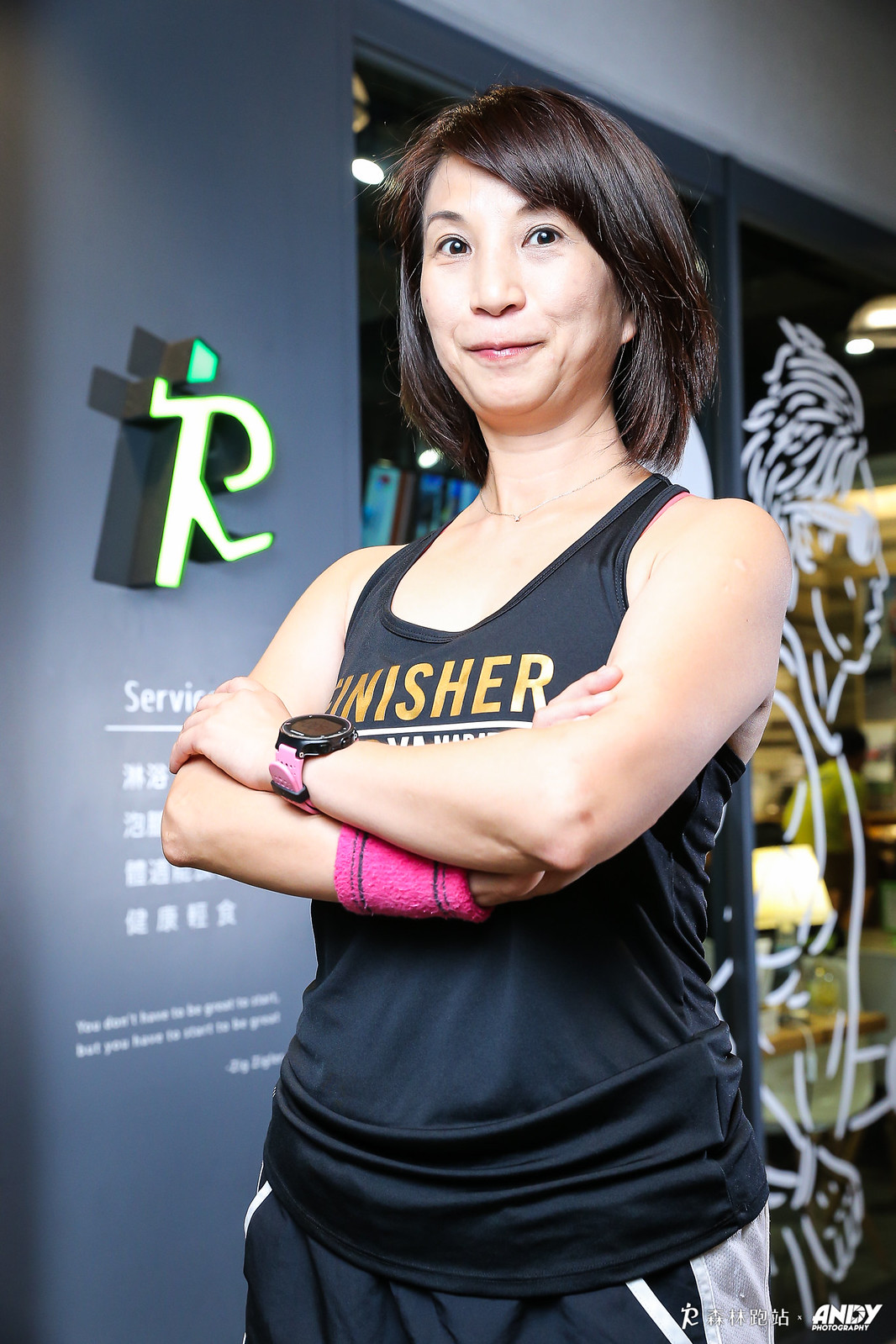The photograph captures an Asian woman with short, straight dark brown hair and bangs, smiling as she stands with her arms folded, her left arm resting above her right. She is clothed in a black tank top with yellow and white text that reads "finisher," along with black and white shorts. On her left wrist, she sports a black-faced watch with a pink band, and on her right, a pink and black wristband. The backdrop consists of dark gray walls, featuring a prominent green neon sign with white text and some Chinese characters underneath. There are glass sliding doors next to the wall, reflecting yellow room lights and adorned with white, edged drawings of a face and hair. The setting suggests she might be inside a gym or fitness area, possibly having just completed a race, as indicated by her attire and the text on her tank top.